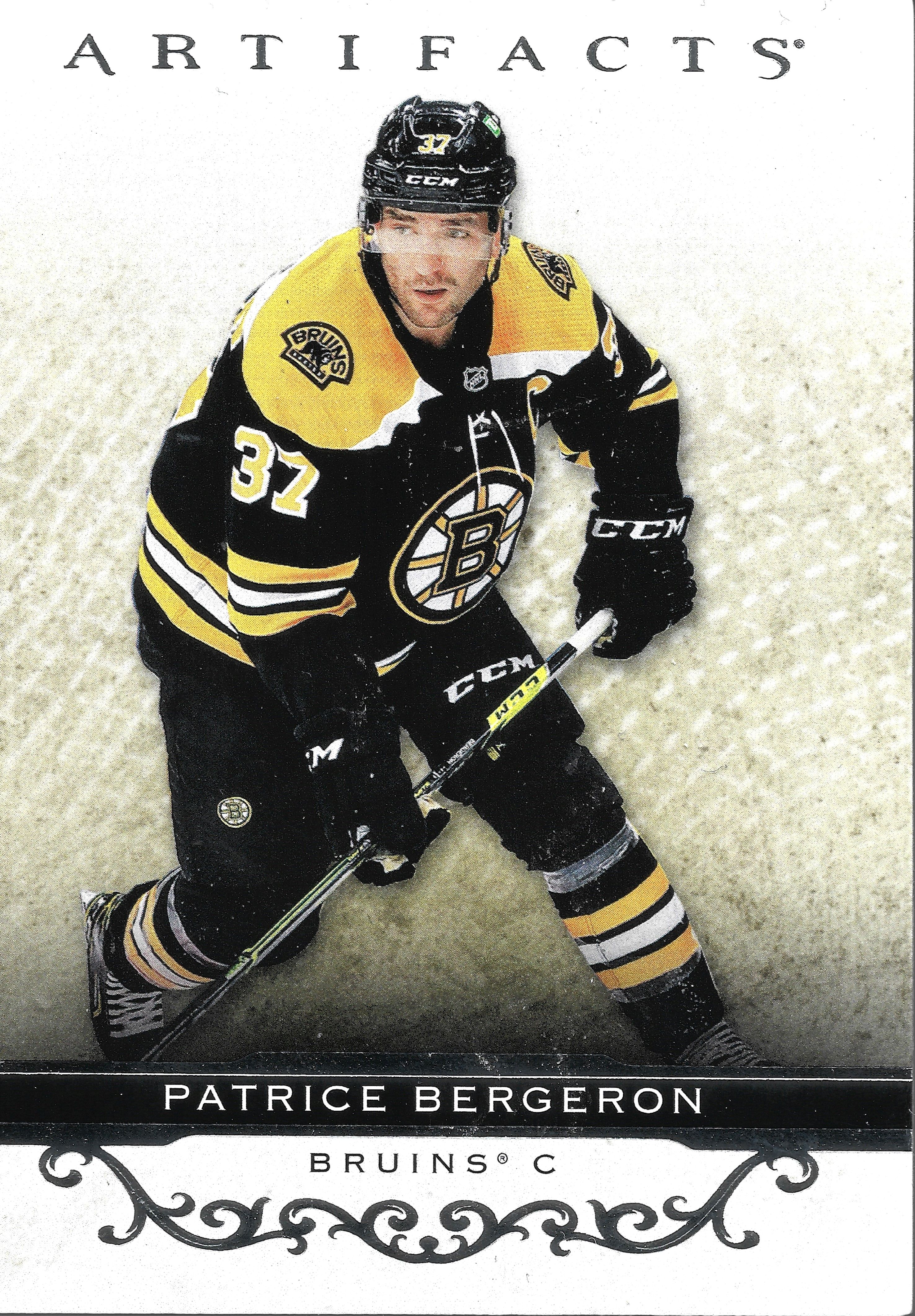This professionally designed collectible card features a detailed, action-oriented photograph of hockey player Patrice Bergeron, who plays as a center for the Boston Bruins. Prominently labeled "Artifacts," the card depicts Bergeron in mid-movement against a plain black, green, and white background. He wears the Bruins' distinctive black, white, and yellow jersey bearing the team logo, his number 37, and bulky protective gear, including a black helmet marked with his number. He is shown holding a hockey stick, with knees bent and wearing thick hockey gloves, long pants, and skates. An intricate, ornate design sits beneath the team name "Bruins," which also features a small copyright logo above the "S." The top of the card displays the word "Artifacts," while the bottom showcases the player’s name, Patrice Bergeron.